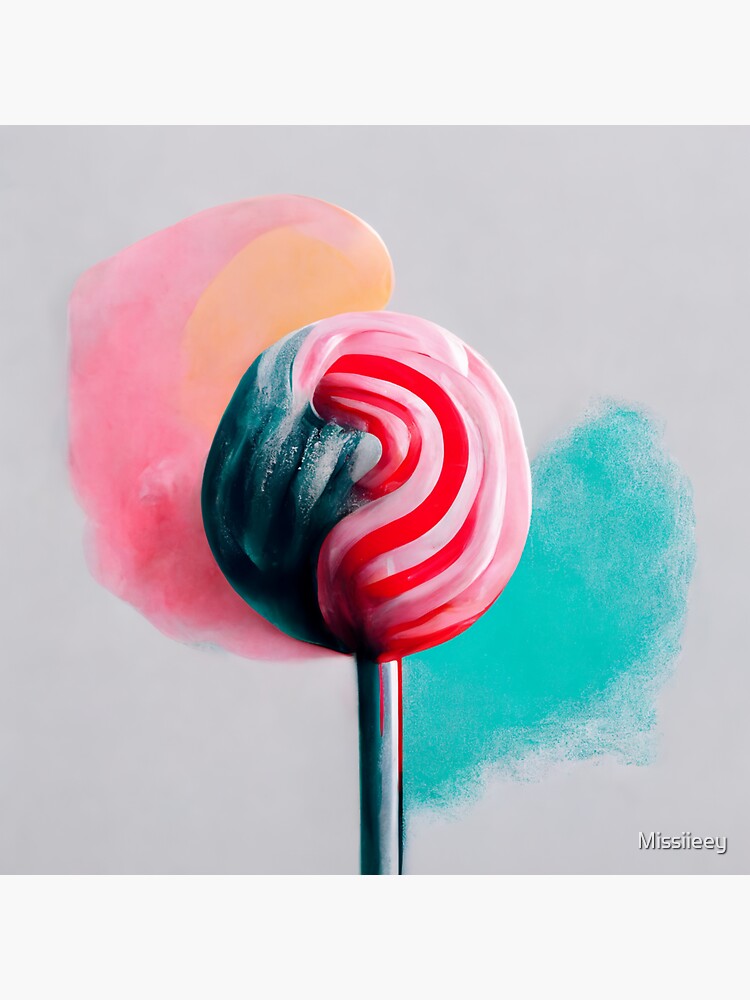This image is a detailed piece of artwork featuring a vibrant, red and blue lollipop with intricately designed cotton candy edges. Set against a bright grayish-white background, the lollipop is centered with a silver or white stem. The lollipop itself is split into two primary colors: the left side is blue with swirling shades of lighter and darker blues, while the right side is pink with a mix of red swirls. Surrounding the lollipop, the left edge has an orange and pink blob suggesting melting candy, while the right side displays a striking bright blue streak. The lollipop's unique design evokes a flag pattern and gives it a realistic, evocative appearance. At the bottom of the lollipop is an inscription, "miss ie," indicating its creator. The cotton candy edges on the lollipop also appear heart-shaped when seen together, adding a whimsical touch to the overall aesthetic.